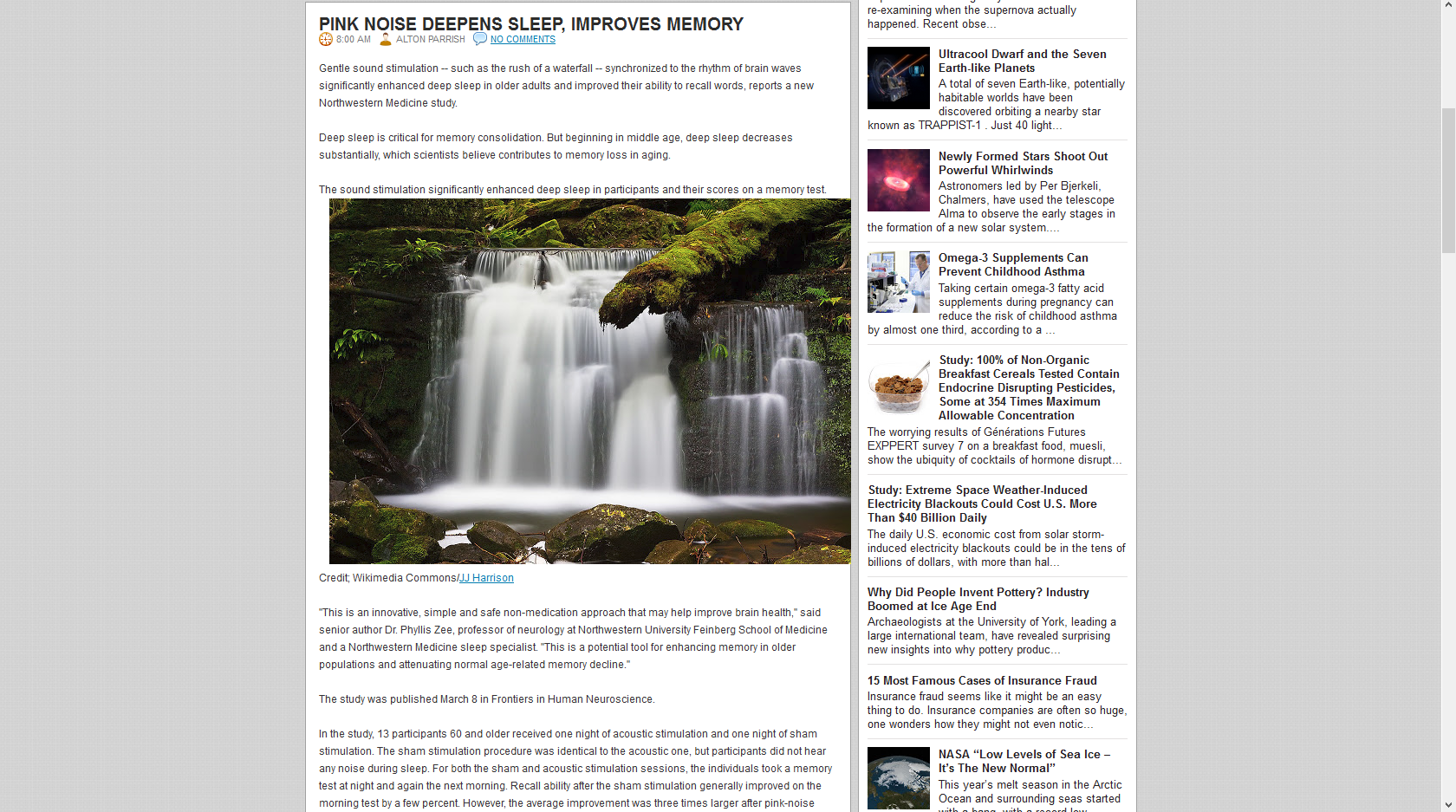This screen capture from a website features an article titled "Pink Noise Deepens Sleep, Improves Memory." The beginning of the article text discusses the benefits of sound stimulation. Dominating the screen is a captivating photograph of an idyllic waterfall. The waterfall cascades over a series of rock formations, with water plunging from various heights—some high and tumultuous, rendering patches of the water foamy white, while others lower and more gentle, creating lighter gray streams. The water collects in a serene pond at the base of the falls. The scene is enveloped by a lush forest, with towering trees and rocks cloaked in vibrant green moss, adding to the tranquil ambiance. The entire setting exudes calmness and solitude, seemingly untouched by human presence. The waterfall, positioned centrally, serves as the focal point of this peaceful, nature-filled landscape.